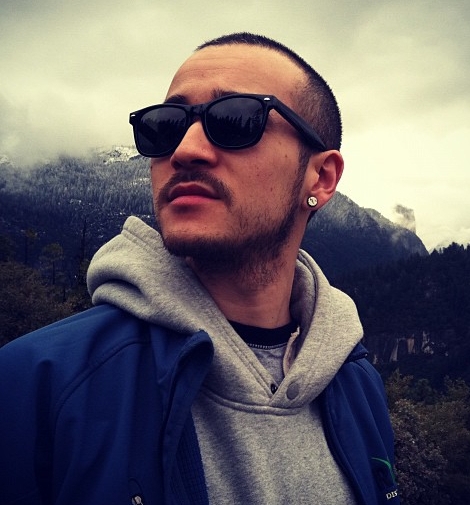This photograph captures a young man, likely in his mid-twenties, against an overcast mountainous backdrop. He has short-cropped dark hair, a black mustache, and a dark but neatly trimmed beard and sideburns that connect. He is wearing Wayfarer-style black sunglasses and sports a large diamond stud in his left ear. His attire includes a black ring-neck t-shirt layered under a gray hoodie, which itself is beneath a royal blue jacket. The image, taken in a three-quarter profile with the man looking to his right, showcases his scruffy facial hair and closely cropped hairstyle. The background features a cloud-covered mountain and forested hills in a Gaussian blur, suggesting a misty day in a natural setting, possibly a national park.